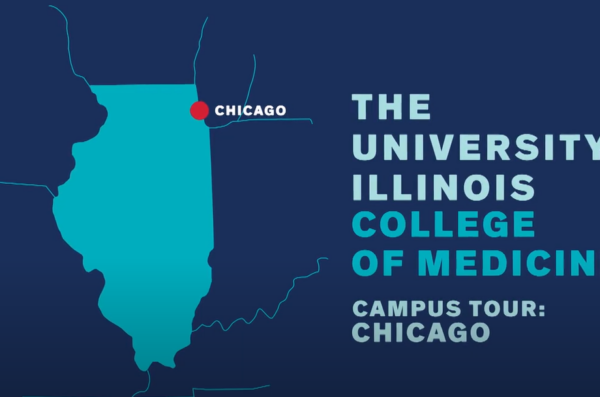This is an advertisement for the University of Illinois College of Medicine, featuring a prominently displayed map of the state of Illinois. The rectangular image primarily comprises varying shades of blue, with the background in a dark blue hue. The map itself is lighter in color, contrasting with the backdrop. A red dot marks the location of Chicago on the top right corner of the map. Bordering states, including Indiana and parts of Michigan, are also visible.

Bold, light blue text overlay reads, "The University of Illinois College of Medicine," matching the color of the state map. Additional text in the lightest blue shade announces, "Campus Tour, Chicago."